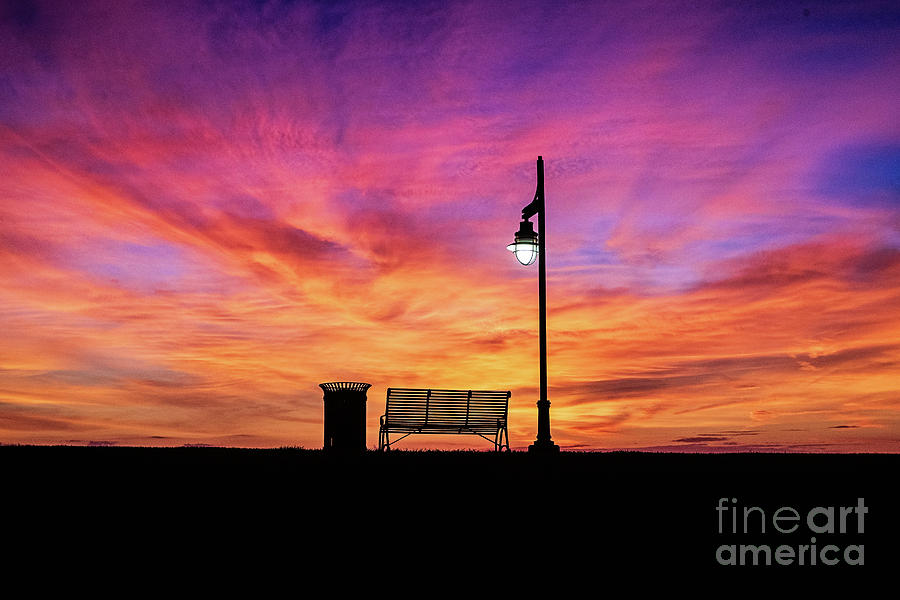This striking photograph captures the vibrant transition of a sunset, framed from a vantage point behind a park bench. The composition prominently features a trash can to the left and a single, illuminated streetlight to the right of the bench. The bottom portion of the image is cast in deep shadow, forming silhouettes of the grass, bench, trash can, and streetlight, which contrasts starkly with the radiant sky above. The sky itself bursts with an ethereal mix of colors—golden yellows at the horizon melding into vivid pinks, deep oranges, purples, and hints of blue, all beneath a dreamy gauzy layer of clouds. The overall effect is both serene and otherworldly. A subtle touch of white light emanates from the street lamp, adding depth and focus. In the bottom right corner, the photograph is marked with the text "Fine Art America," signifying its artistic value.